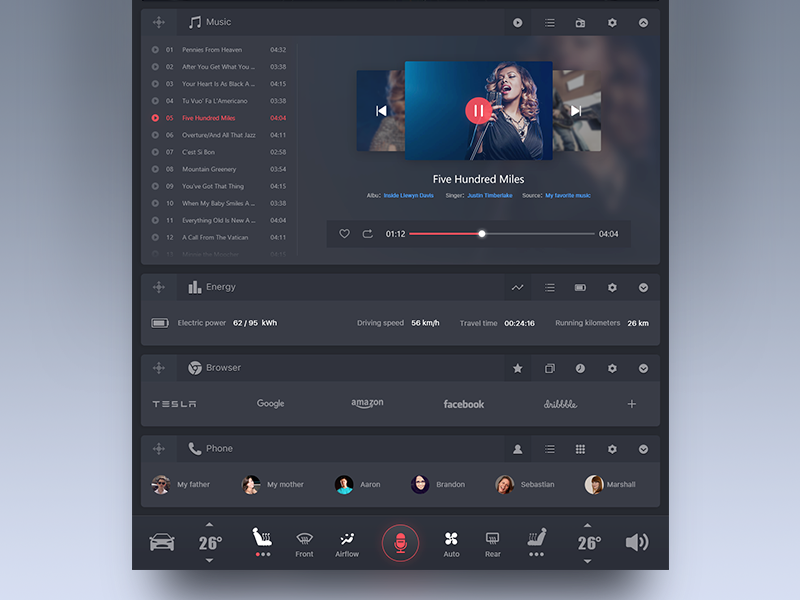The image is a screenshot of a music application interface. At the top left corner, the app title "Music" is prominently displayed. Below this, there appears to be an album cover, although the details are somewhat blurry and hard to discern. On the right side of the screen, there is a picture of a woman who seems to be singing, her image bathed in a soft focus. Beneath her photo, the title of the current track, "500 Miles," is clearly written in bold white font. A progress bar shows that the song is at 1:12, with a total duration of 4:04. Beneath this interface, there are sections labeled "Energy," "Browser," and "Phone," suggesting additional functional categories within the app.